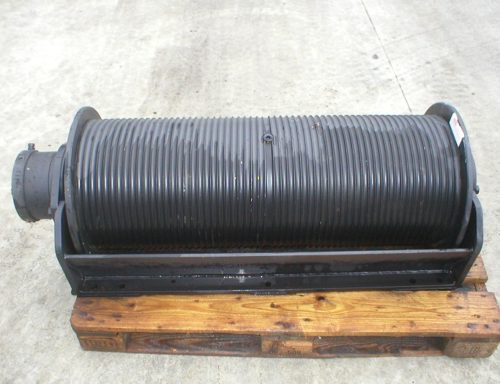The image depicts a mechanical object with an uncertain purpose, resembling a cylindrical tool or gadget. This object, predominantly black with intricate grooves running horizontally, is metallic in nature. Its left end features a cast iron-colored attachment point, extending a few inches, suggesting it can be connected to another component. Positioned on a rich, dark brown wooden pallet, the object contrasts sharply with its backdrop. The pallet rests on a white or light gray tiled or concrete floor, indicating a workshop or garage setting. Notably, on the right side of the cylinder, there is a white rectangular tag attached to its inner edge, possibly a price sticker or identification label.